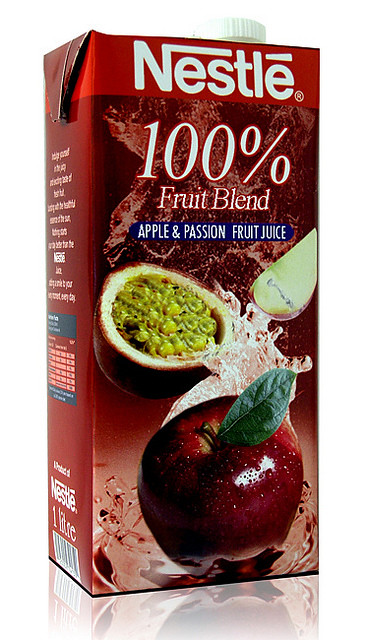The image depicts a digitally rendered Nestle juice carton, prominently featuring a vibrant red design. At the top, below a white screw cap, the Nestle logo is displayed in white lettering with artistic flourishes. The text "100% fruit blend" is outlined in red, indicating the purity of the fruit content. The main label reads "apple and passion fruit juice" inside a dark blue rectangle filled with white text.

The central visual showcases a red apple with a green leaf, partially submerged in clear, splashing water, adding a refreshing dynamic to the imagery. Adjacent to the apple is a sliced-open passion fruit, revealing its juicy, green interior bordered by a beige rim. The right side of the box reveals a piece of the apple seemingly flying to the right, adding a sense of motion.

Reflections and shadows have been digitally applied to enhance the three-dimensional look of the carton, with folded corners producing a triangular maroon-red effect. Although part of the left panel’s nutritional information and a barcode are visible, specific details remain unreadable. This image portrays an adult-oriented juice carton, holding one liter of the fruit beverage, encapsulating both artistic design and clear product information.